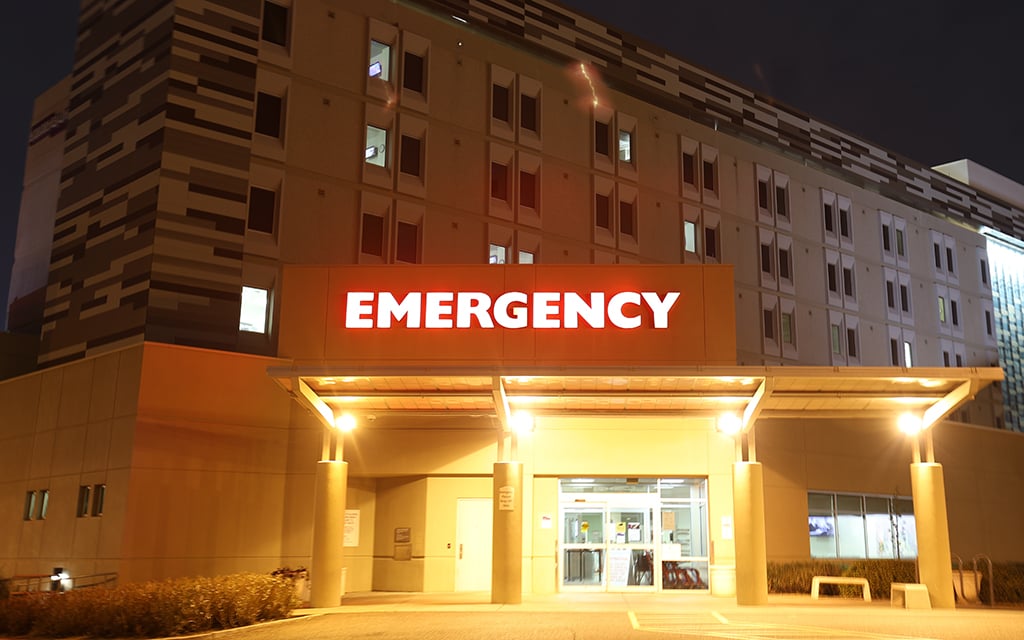This photograph captures the entrance to a hospital's emergency room at night. In the foreground, a portion of the parking lot is visible, bordered by green hedges on the left. The lower section of the hospital building is a tan color and features four posts supporting an awning. The awning is brightly illuminated, casting a yellow glow over the entrance area. The glass windows and doors of the emergency room entrance are clearly visible. Above the entrance, there is a tan sign with bold, illuminated red lettering spelling out "EMERGENCY." In the background, the hospital building rises to four floors, with a mix of lit and unlit windows. The building exhibits a tan, gray, and black pattern on its facade.